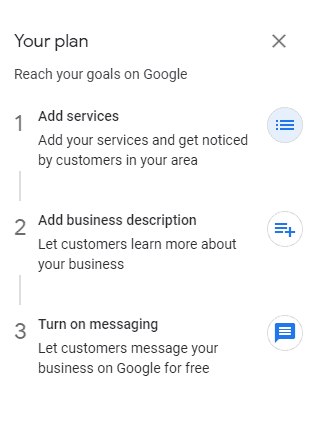In this informative graphic, a white background provides clarity for viewers. Step-by-step instructions guide users on how to improve their local business presence on Google.

1. **Add Services**: The first section prompts users to enhance their business profile by adding services, allowing potential customers to easily discover what they offer. This is illustrated with an 'X' symbol on Google, aiding in emphasizing the importance of this feature.

2. **Add Business Description**: The second part highlights the need to provide a detailed business description. This enables customers to gain deeper insights into the business. This step is visually represented by a circle containing three squares, each square adjacent to three rectangles, symbolizing text details.

3. **Turn on Messaging**: The final step encourages businesses to activate messaging, facilitating direct communication with customers via Google for free. This feature is depicted by a circle containing a blue chat icon, adorned with three white lines or rectangles, representing text messages.

This comprehensive image ensures businesses know how to optimize their presence and interact efficiently with their local customer base.